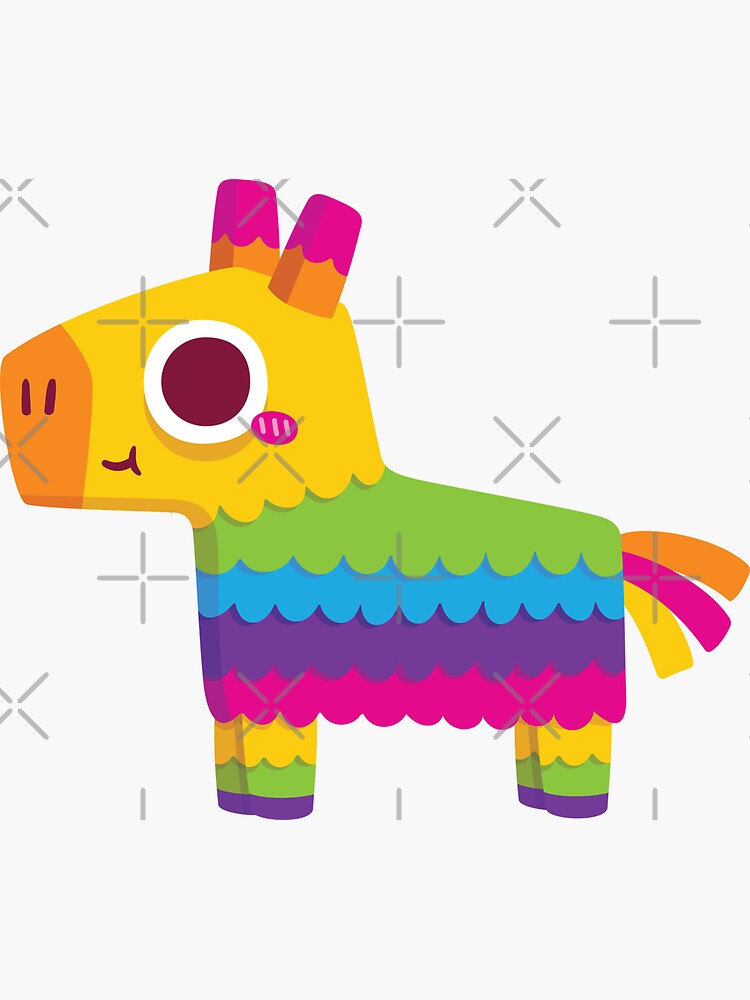This digital illustration captures a vibrant, multi-colored piñata shaped like a horse, set against a light green background adorned with gray X's and plus signs. The horse's head is predominantly yellow, featuring a large brown eye surrounded by white, and decorated with pink spots and a gentle smile. Its rectangular ears resemble popsicles with an orange base transitioning to pink. The orange nose is accented with dark pink nostrils. The piñata's body displays a scalloped pattern of colorful stripes: green at the top, followed by layers of light blue, purple, and pink. The flamboyant tail consists of feather-like strands in orange, yellow, and pink. The legs combine yellow, green, and purple hues, ending in purple hooves. This whimsical, rainbow-colored piñata exudes a playful and child-friendly charm, making it perfect for children's stationery or festive designs.